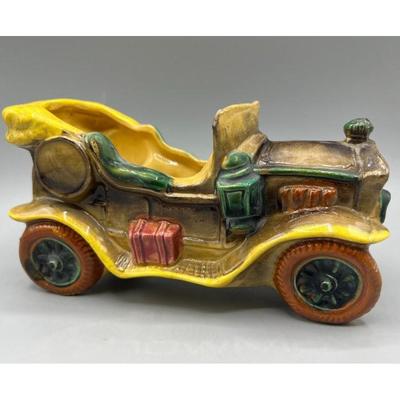The image captures a detailed vintage ceramic convertible car, meticulously crafted and likely handmade from clay. The model appears to echo an old-style 1920s Ford Model T Roadster. The car, facing the right side, features a glossy, glazed finish with a predominantly mustard yellow exterior and brown-yellow sides. The interior holds yellow seats, emphasizing the open two-seater design, lacking a roof. Visible from the front are two orange rubber wheels, accented with dark green rims. A quaint reddish-brown box is affixed to the car's side, accompanied by a green-painted lantern near the handle, adding to its nostalgic charm. The entire scene is set against a white background, enhancing the car's intricate artistry.